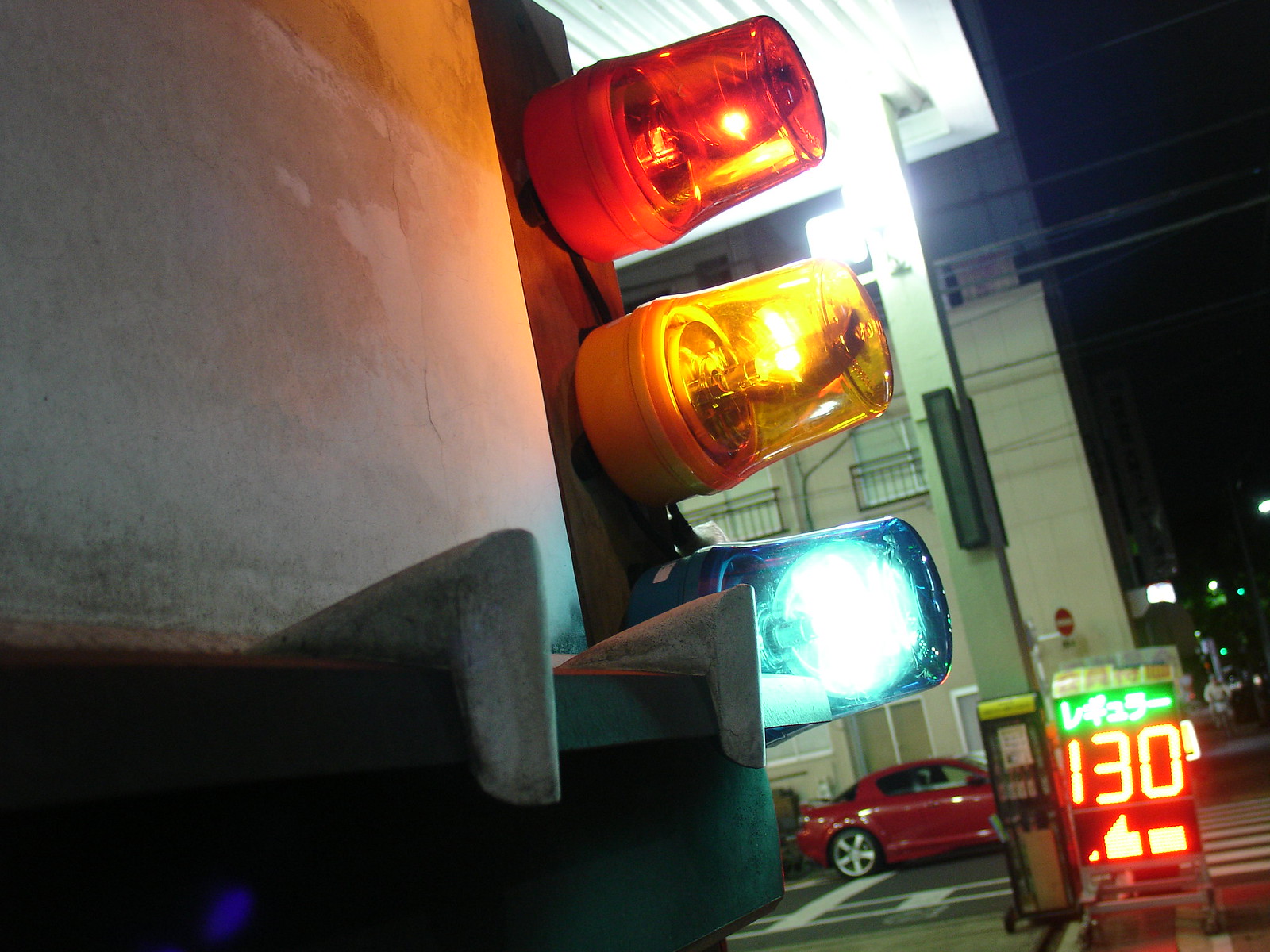The image features three emergency stoplights, mounted vertically on a black wall, extending outward without protective covers. The top light glows red, the middle one yellow, and the bottom one blue, all facing towards the upper right. To the right and slightly below these lights is a digital sign displaying the number "130" in red letters, with an additional glowing white arrow outlined in green. In the background, a red sports car is parked on the street, accompanied by white crosswalk lines. This street scene is set against a tan building with gold-colored metal barriers on its windows. The night sky is pitch black, enhancing the illuminated elements and the urban setting.